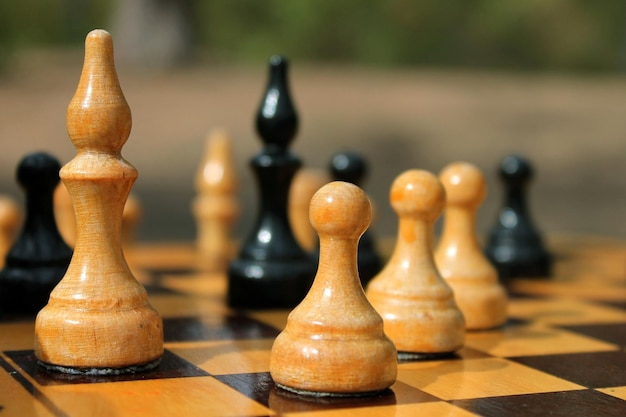The image is a macro photograph capturing a detailed and close-up view of a polished, wooden chessboard with tan and dark brown squares. In the foreground, the focus is sharply on three tan pawns aligned on black squares, drawing immediate attention to their pristine, wooden texture. Beside them is a larger tan piece, likely a bishop, also in clear focus. The background of the image displays a blurred green and tan hue, suggesting an outdoor setting with possibly blurred trees. Additionally, the out-of-focus background features shiny, standard black chess pieces, including another bishop and a black pawn, creating a smooth gradient of blur. The photograph is taken from an angle, enhancing the depth and lending an artistic lens blur effect that accentuates the crisp details of the white pieces in the foreground while subtly hinting at the numerous black pieces, at least ten, scattered throughout the board.